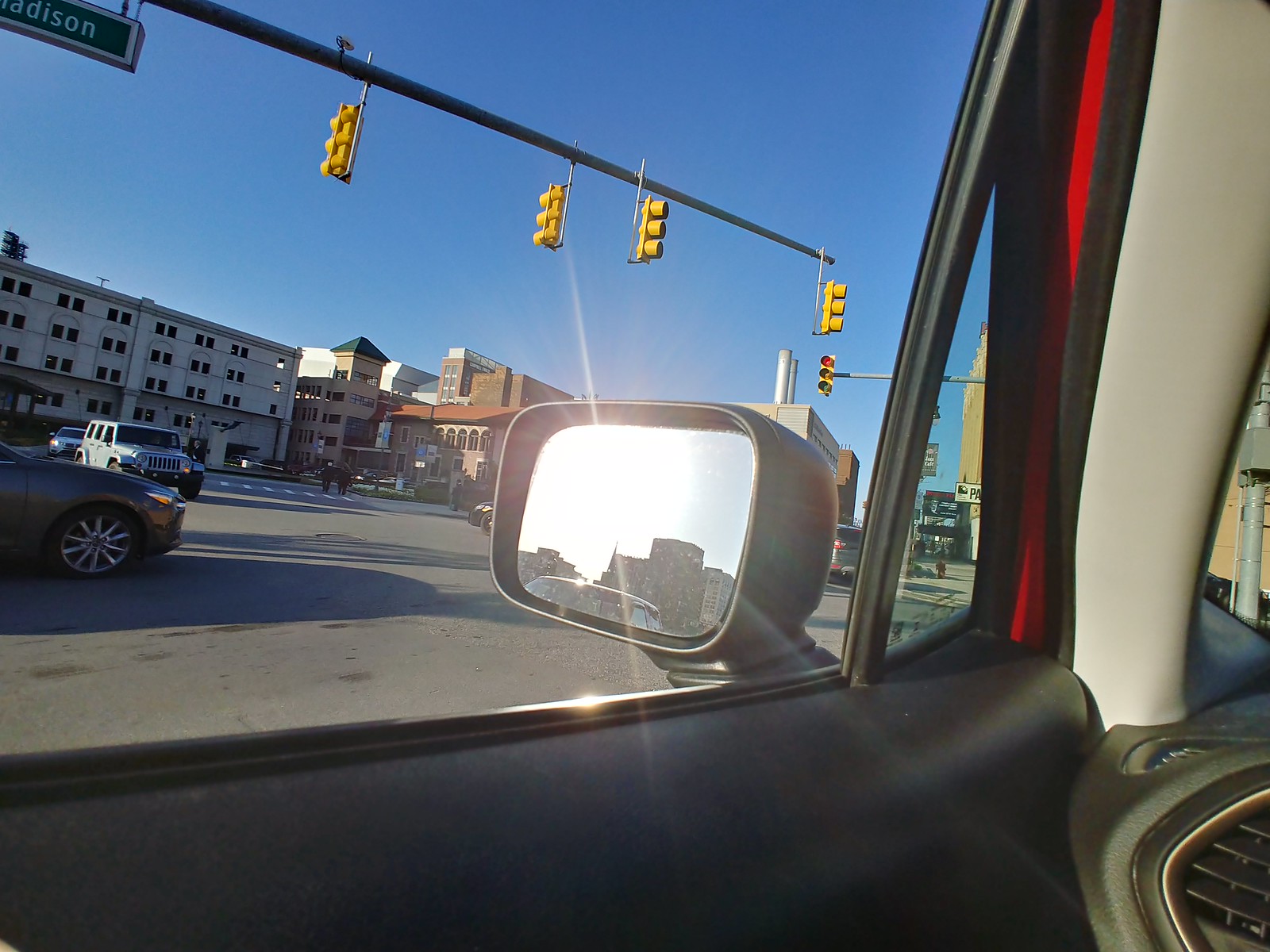The photograph masterfully captures a bustling urban intersection, juxtaposed with its reflection in a car's rearview mirror, creating a dynamic and well-choreographed scene. Traffic signals are prominently suspended over the intersection, held aloft by arms and booms, all set against a crisp blue sky. The backdrop features an array of modern buildings, including residential units and business complexes. Central to the image is a parking area adorned with a multi-level ramp and a towering elevator structure at its summit. To the right, one can observe the imposing silhouettes of smokestacks belonging to a nearby power plant.

Views through the car window offer an additional layer to the composition, where the rearview mirror reflects more urban landscapes, including multi-story buildings that are not exceedingly tall but stretch several floors high. The entire scene, inclusive of the live intersection, the rearview mirror reflection, and the distant buildings beyond the traffic lights, paints a vivid and detailed portrayal of a bustling cityscape.